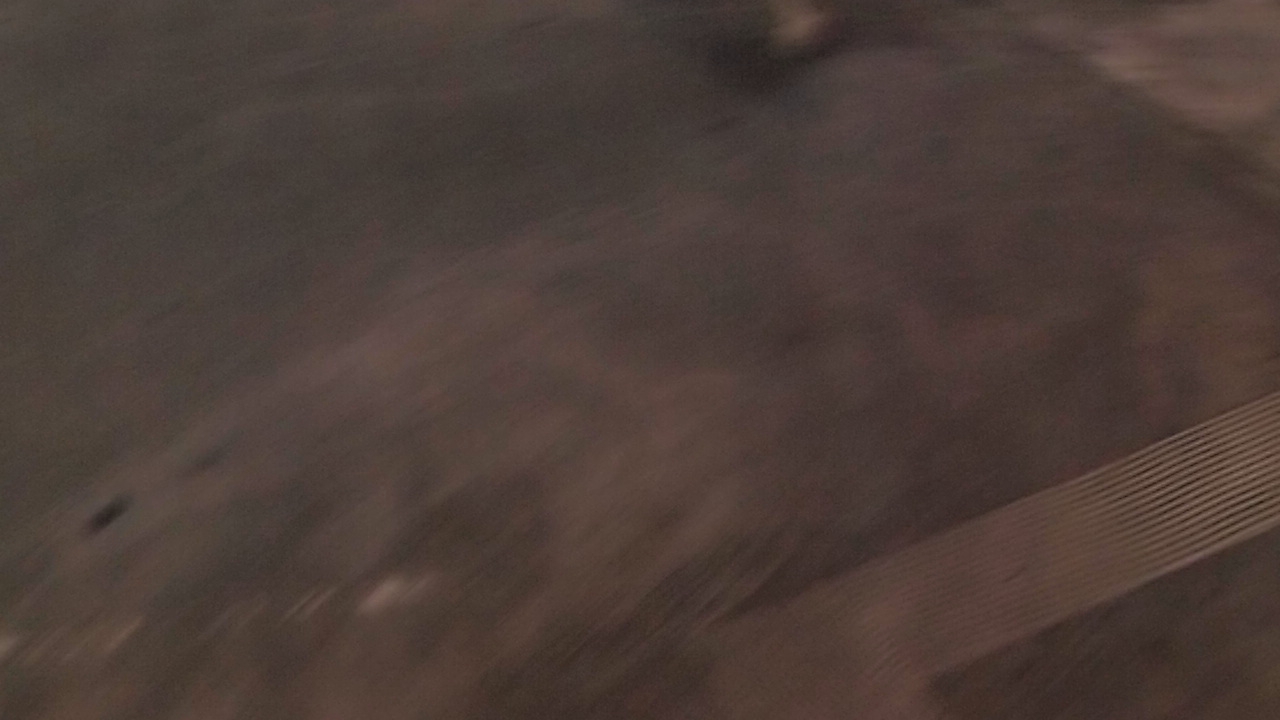The image is predominantly a blur with indistinct features, giving it a brownish hue. Diagonally, from the right-hand side and about two-thirds of the way down, there are some vague white lines that seem to fade away as they move downward. The rest of the image appears muddled with various shades and lacks clear definition. On the lower left-hand side, there are small white patches resembling brush strokes, and above these, there's a dark area that vaguely resembles a nose. Towards the top of the image, there are both a dark spot and a small white spot. Overall, the image remains ambiguous, possibly a close-up of an indeterminate subject.